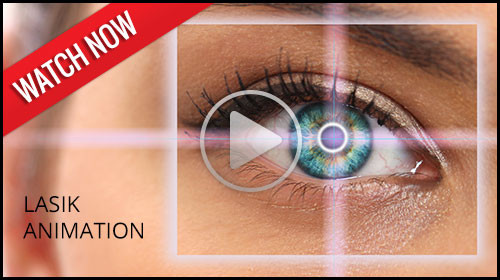This image appears to be a digitally enhanced photograph, likely used as a video advertisement for LASIK surgery from a company called LASIK Animation. The focal point of the image is a detailed, realistic eye that dominates the center-right side of the frame. The eye itself has a rich, blue base with remarkable shades of yellow, and possibly hints of turquoise-green. It features long black eyelashes and appears to belong to a female with brown eyebrows. The eye is enhanced with makeup to accentuate its allure.

The image includes various visual elements indicative of an interactive video advertisement. At the center of the eye, there are a translucent white play button and a crosshair formed by thin white lines, highlighting the focus of the LASIK procedure. A clear square outlines the eye, making everything outside of it blurry, drawing attention to the eye itself.

In terms of text, a red banner in the upper left corner reads "watch now," and there is thin black text in the lower left corner that says "LASIK Animation." The entire image is enclosed with a very thin black border, adding to its polished appearance. The dimensions of the image are approximately 3 by 2 inches. Overall, the image is a cleverly designed advertisement meant to engage viewers and entice them to watch an animation explaining LASIK eye surgery.